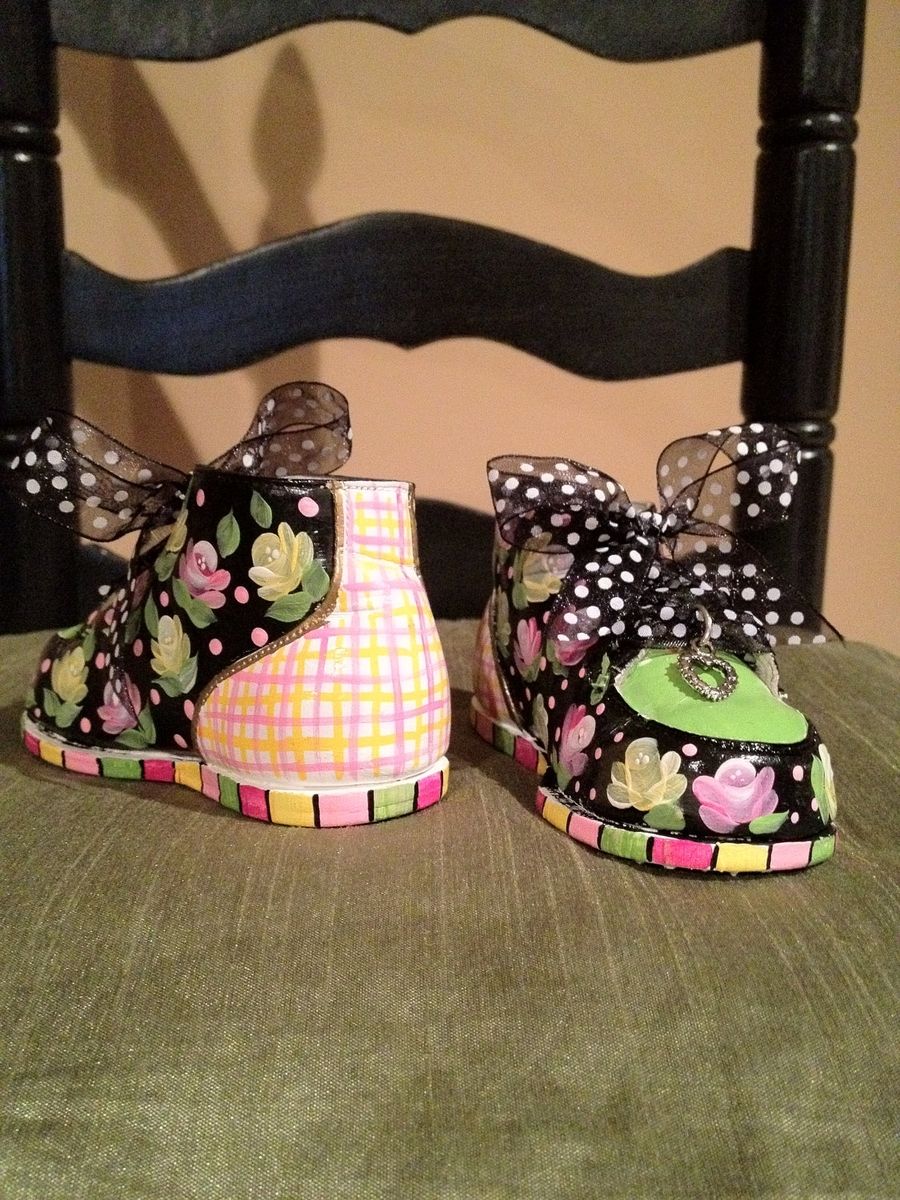The photograph captures a pair of small, decorative porcelain or ceramic shoes, intricately painted with vibrant patterns including roses, polka dots, and stripes in colors like yellow, red, pink, and green. These shoes, which appear hand-painted, feature sheer mesh and black ribbons with white polka dots as laces, accented by heart charms. One shoe faces towards the viewer while the other faces away, showcasing a pink and yellow plaid pattern on the back. They rest on a chair with an olive green fabric seat, which has a black-painted wooden frame. The setup casts a shadow on the pale salmon peach-colored wall in the background, further enhancing the amateur quality of the image.